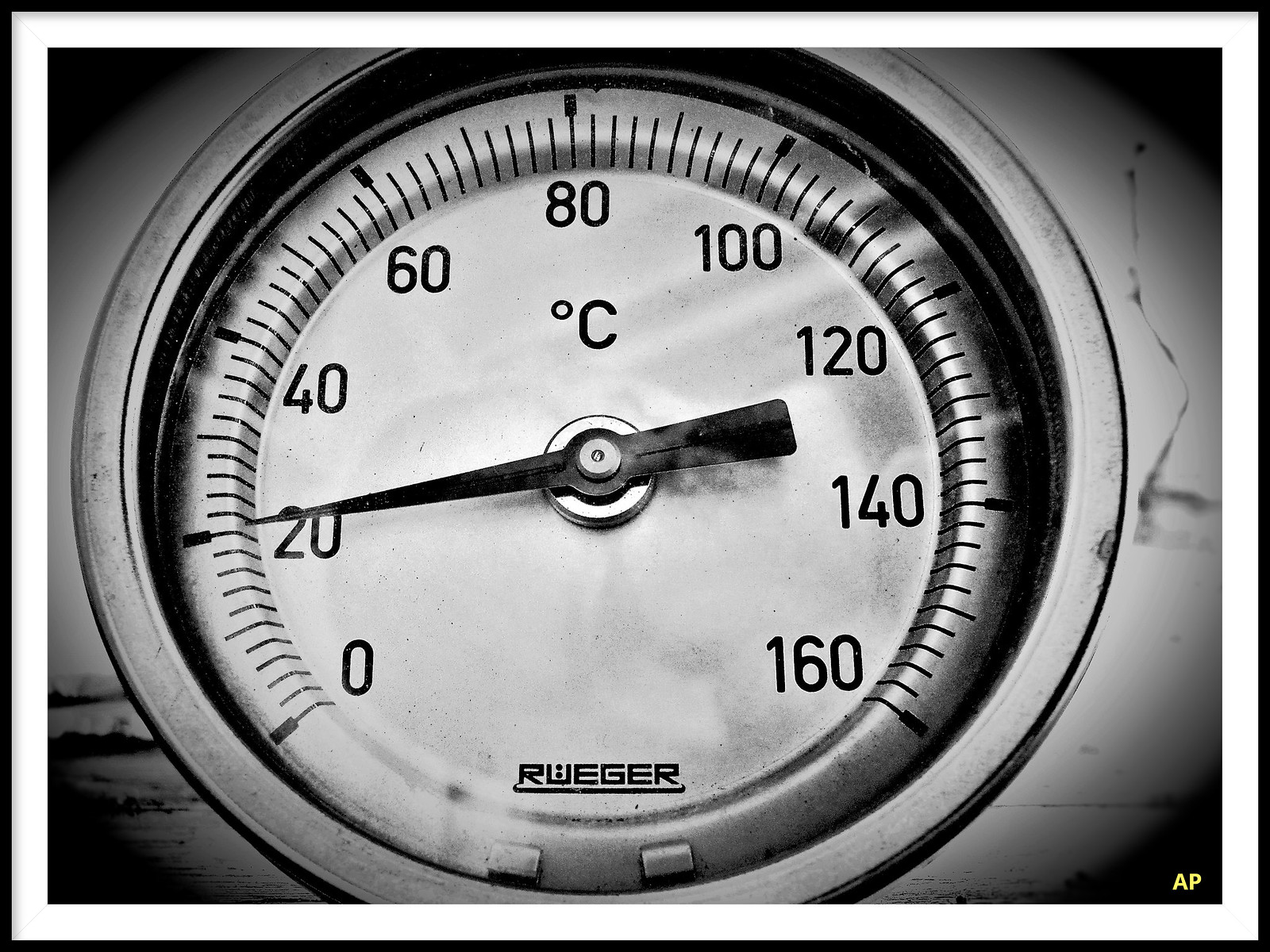A black and white photograph captures a vintage, round gauge, which appears to be made of silver. The dial prominently displays the brand name "R-W-E-G-E-R" at the bottom, with a line beneath it. The gauge features a numeric scale that starts at 0 on the left side and progresses clockwise to 160 on the right. The 0 to 40 range and the 120 to 160 range are marked with numerals, while the bottom segment remains unnumbered. Precise lines indicating increments of two are etched between the numbers along the scale. A black arrow-shaped needle points leftward to the number 20. Above the needle and just below the number 80, there is a symbol denoting degrees Celsius. The gauge rests against a subtly shadowed, gray background, but the absence of any reference objects makes it difficult to gauge its exact size.